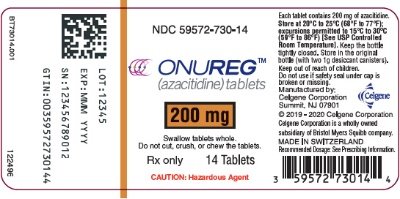In this image, the back of a pharmaceutical tablet package is prominently displayed against a red background. The product is identified as a CitiDyne tablet, bearing the lot number 12345 and a serial number 123456789012. An expiration date is also noted. To the left of the tablet package, a QR code is visible, accompanied by the alphanumeric identifier BT730014001 below it. On the right side of the QR code, the text 12249E is printed. The tablet packaging also includes a label specifying the contents: each tablet contains 200mg of CitiDyne. The storage instructions advise keeping the tablets at a temperature between 20°C to 25°C.